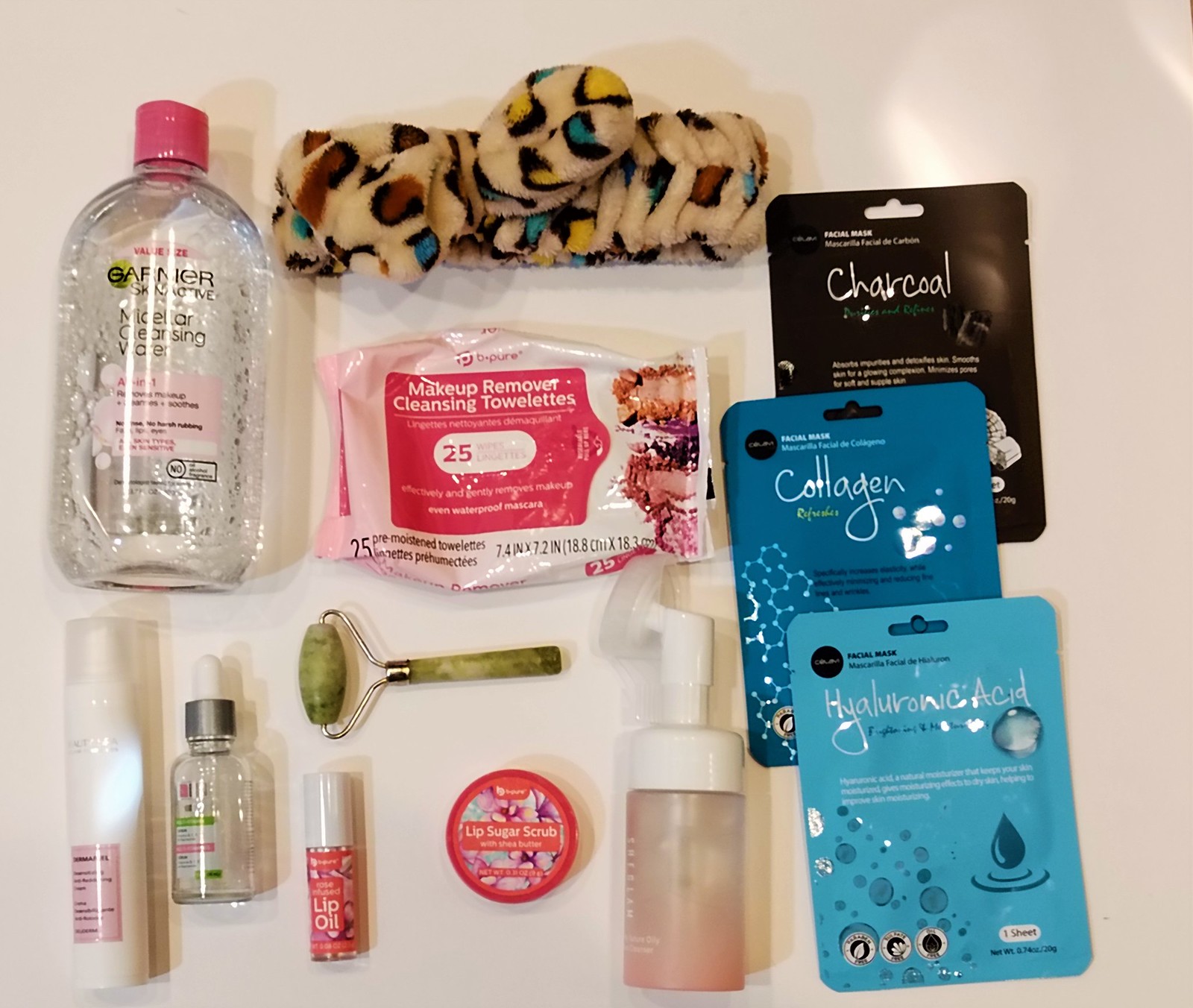The image features an assortment of beauty products neatly arranged on a surface that might be a counter or a wall. On the far left, there is a transparent plastic bottle with a pink cap labeled as some kind of cleansing water, resembling a large baby oil bottle. Below this bottle are two smaller bottles, both equipped with droppers. The one on the left has a transparent cap containing a milky white liquid, while the one on the right holds a clear liquid.

Centrally positioned, from top to bottom, are various items: a hair scrunchie, a packet of makeup remover cleansing towelettes, and a ceramic roller used for muscle relaxation. Adjacent to these, there is a container of lip oil and a lip sugar scrub, followed by a plastic container with a white cap.

On the right side of the arrangement, there are three differently colored packages stacked vertically. The top package is black and labeled "charcoal," the middle one is dark blue and labeled "collagen," and the bottom one is light blue, labeled "hyaluronic acid."